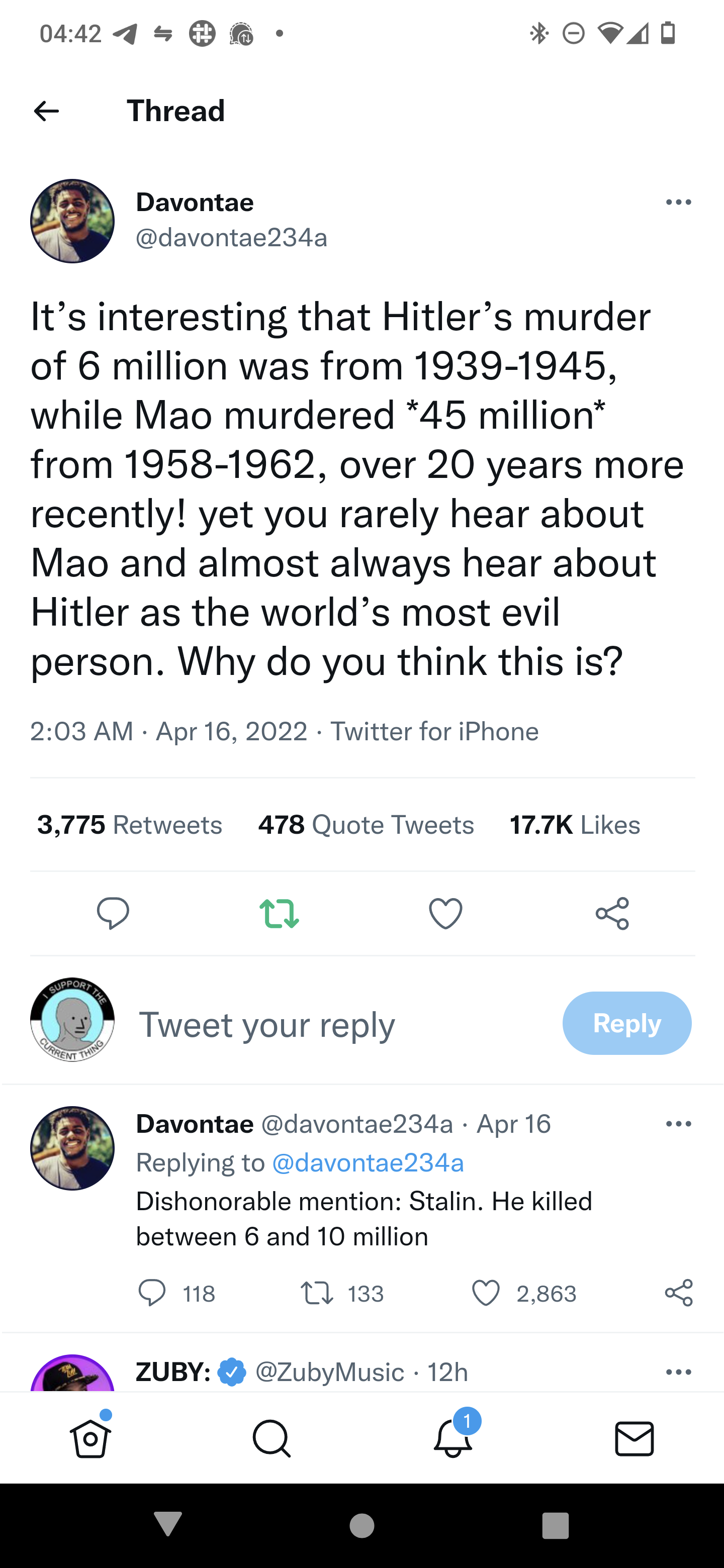The upper part of the image features a white background with the time displayed in gray, indicating 04:42. Adjacent to the time is a rightward-pointing arrow accompanied by two half-arrows in opposite directions. Below this, there is a gray circle intersected by white lines, followed by two gray text boxes. One of these text boxes contains up and down arrows, while the next features a small gray circle with indeterminate symbols, including triangles and lines. Further down, a white circle with a gray outline and a gray dash is visible, along with a gray Wi-Fi icon indicating good reception. The battery icon suggests a charge level of less than 30%.

The main content consists of black text starting with a name, "Devante," beside a circle showing a profile picture of a smiling black male wearing a black shirt. Below, "Devante, 23, 4A" is stated, followed by three black dots on either side of the next segments of text. The text reads:

- "Interprets as a Hitler's murders that murdered 6 million was from 1939 through 1945."
- "While Mao murdered 45 million with two extras on each side."
- "From 1958 through 1962, over 20 years more."
- "Recently, yet you really hear about;"
- "And almost always hear about;"
- "Hitler as the world's most evil person."
- "Why do you think this is?"

It also references the creation or discovery of the message with "This tool. 3 a.m. April 16, 2002. I found 3,775. 478. Tweets. 17.7K Likes."

The overall structure conveys a comparative statement about historical figures, implying a critique of common perceptions of their notoriety.